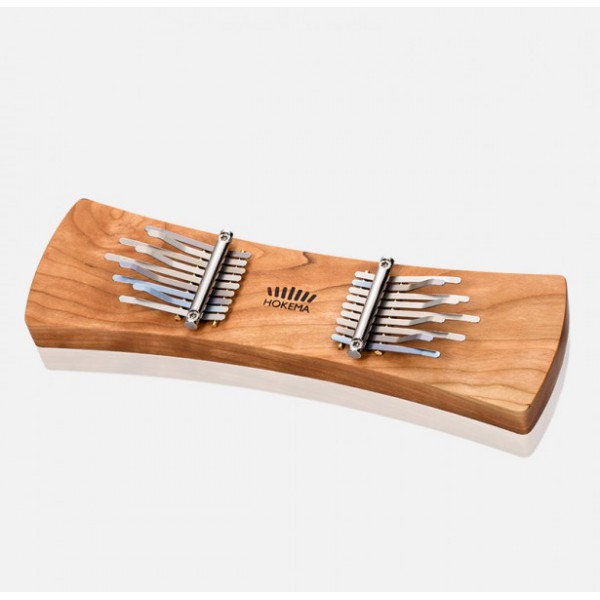This image depicts a small, uniquely-shaped musical instrument with a wooden base. The base, almost rectangular with slightly concave top and bottom edges, has a warm brown color adorned with darker lines. Centered on this wooden base is a black inscription reading "Hokema," above which is a logo comprising seven vertical lines. On either side of the inscription, metallic keys are arranged horizontally, with about six or seven on each side. These silver, horizontal metal strips point outward and upward, resembling keys that can be flicked to produce sound. The instrument is set against a light gray background, accentuating its detailed design and structure.